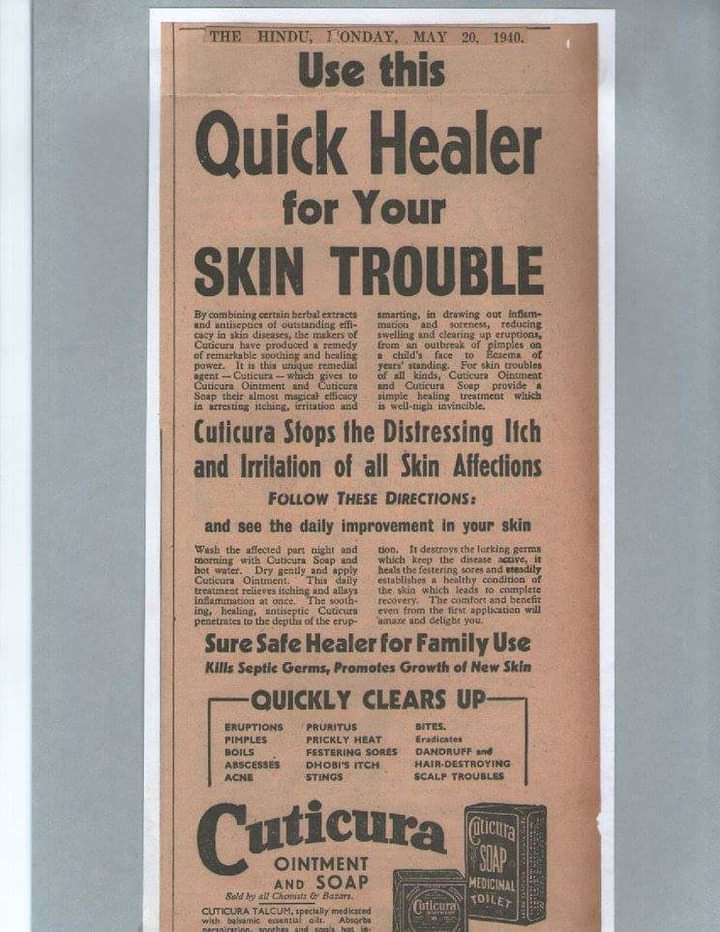This image features an old newspaper clipping that is centrally placed against a solid medium gray background, possibly resembling a sign. The clipping, distinctly aged with a brown background and white border, originates from "The Hindu," dated Monday, May 20th, 1940 (with one incorrect mention of 1946). Dominating the top is a bold black headline: "Use this quick healer for your skin trouble." Below it, arranged in two columns, is the main body text describing the product. 

Further down, a smaller headline reads: "Cuticura stops the distressing itch and irritation of all skin affections," followed by an instruction: "Follow these directions and see the daily improvement on your skin." This section is also arranged in two columns. 

Another heading, "Sure safe healer for family use, kills septic germs, promotes growth of new skin," introduces the next segment. Under it, emphasized with horizontal lines extending from both ends, the text "quickly clears up" precedes a list of skin issues the product alleviates, arranged in three columns. 

At the bottom, in curved, large black bubble letters, is the brand name "Cuticura," followed by "Ointment and soap." Two detailed outlines of Cuticura soap boxes complete the advertisement. This long, vertical ad reflects the typical layout of products in a 1940s Indian newspaper, emphasizing various skin-related benefits.